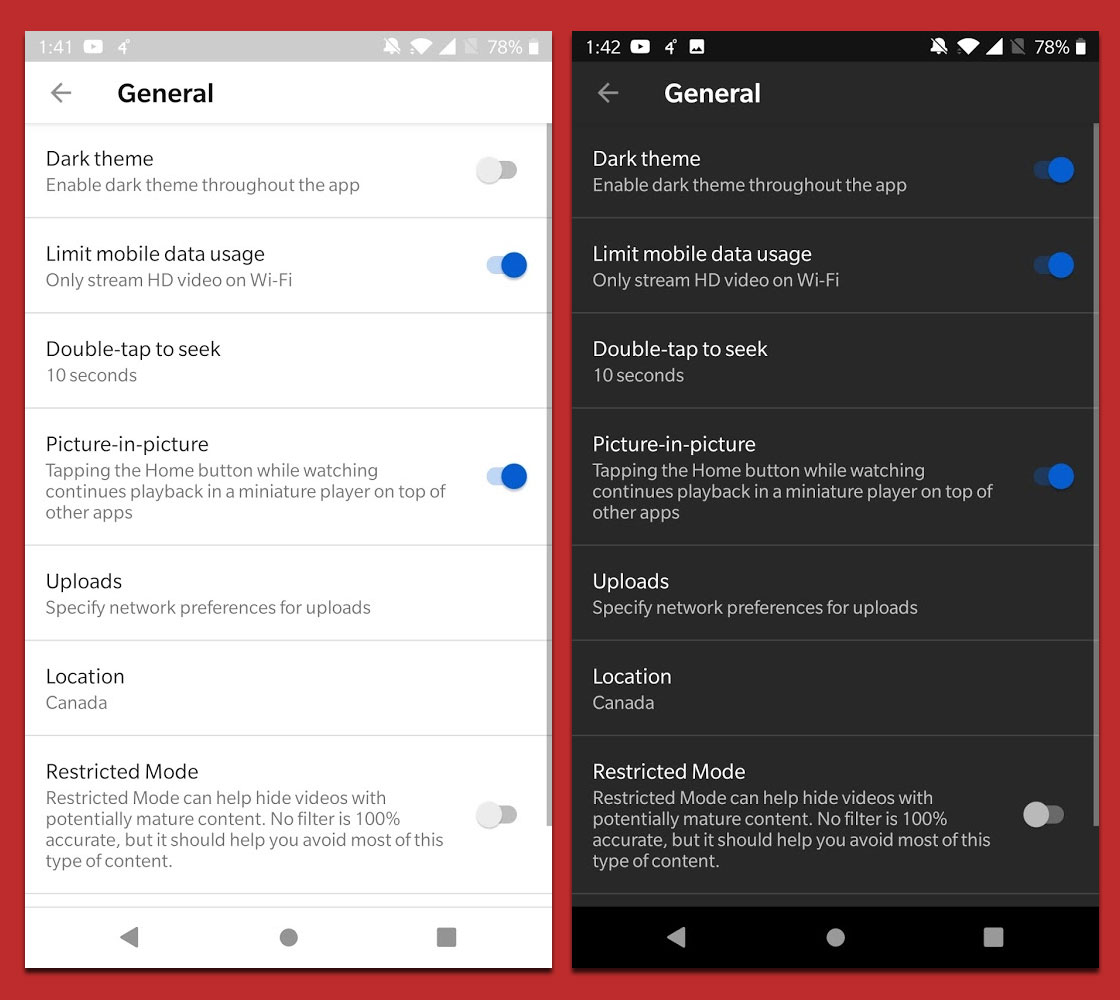A screenshot showcases a mobile device with a split-screen interface, divided vertically by a red line. The screen appears to depict the settings page of an app, featuring both a light theme on the left and a dark theme on the right, demonstrating the theme toggle functionality. 

At the top of the screen, the system time is consistently displayed as 1:41 on the light-themed side and 1:42 on the dark-themed side, with both sections showing a battery life of 78%. The title "General" is prominently displayed under the status bars on both sides.

Each section lists various settings:
1. **Dark Theme**: Both sides include the option "Enable dark theme throughout the app," with the toggle switched to 'On' in the dark-themed section, thereby showing its activated state.
2. **Limit Mobile Data Usage**: This option is turned on in both themes.
3. **Double Tap to Seek**: No slider is shown for this setting.
4. **Picture-in-Picture**: This feature is turned on, indicated by a blue highlight.
5. **Uploads**: No slider available.
6. **Location**: No slider available.
7. **Restricted Mode**: This setting has an available slider but remains off.

The light theme is depicted with a white background and black text, while the dark theme features a black background with white text, emphasizing the contrast and functionality of the app's dark mode.